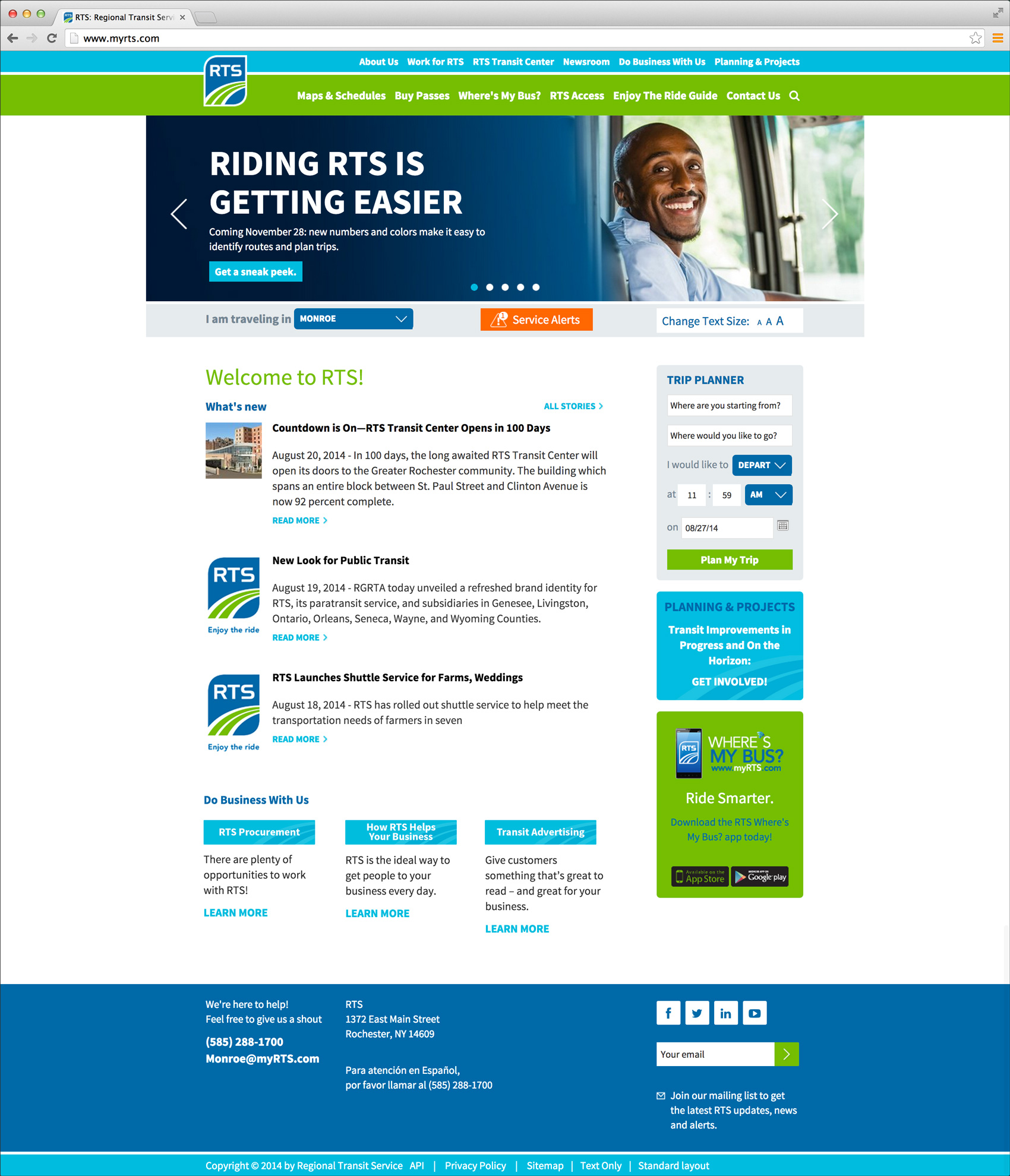The image is a screenshot of the RTS (Regional Transit Service) website. At the very top, there is a gray search bar displaying the URL "www.myrts.com." Just below, a dark gray tab indicates the page is titled "RTS Regional Transit Service."

Below the navigation bar, a thin, baby blue horizontal menu features several tabs: "About Us," "Work for RTS," "RTS Transit Center," "Newsroom," "Do Business With Us," "Planning and Projects." 

Further down, a green strip contains additional options: "Maps and Schedules," "Bus Passes," "Where's My Bus," "RTS Access," "Enjoy the Ride Guide," and "Contact Us."

Dominating the main section of the page is an image of a bus driver. The driver is a bald, dark-skinned man with a beard and mustache, wearing a pale blue shirt. The bus driver appears to be in motion, as he's seen operating the bus. Superimposed on the image, a message reads: "Riding RTS is getting easier. Coming November 28, new numbers and colors make it easy to identify routes and plan trips." Below this message, there is a blue button labeled "Get a Sneak Peek."

Following this, there is a section with a blue drop-down menu titled "I am traveling in" where the current selection is "Monroe," and an orange button labeled "Service Alerts and Change Text Size AAA."

At the very bottom, in green text, the website welcomes visitors with the message: "Welcome to RTS."